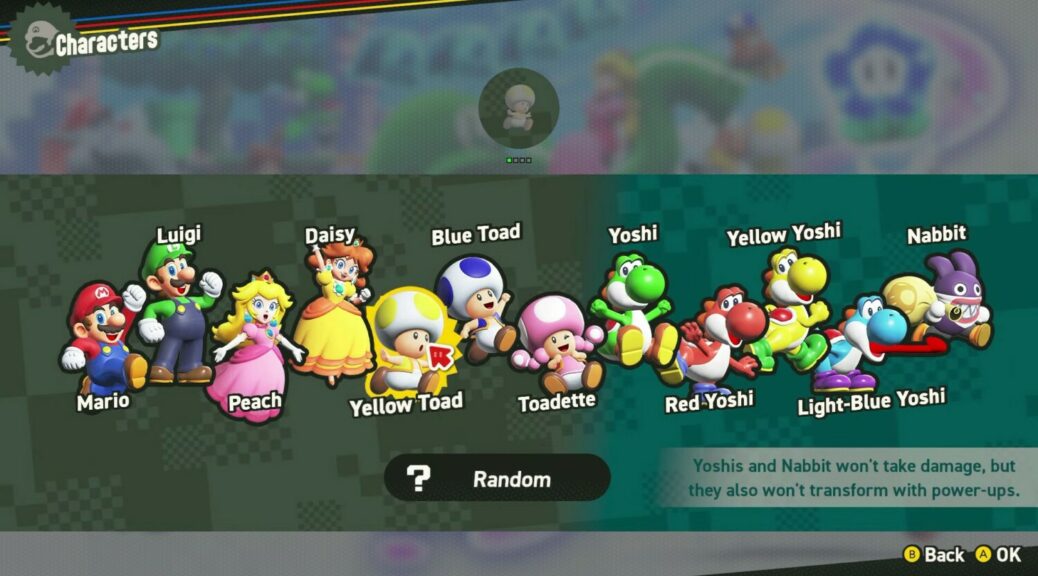The image appears to be a screenshot of a Mario-themed video game character selection screen, likely from a Nintendo game. The layout is horizontal and rectangular, set against a dark green background. At the top left corner, white text reads "Characters," under which various character icons are arranged. Each character is labeled with their name in white text. From left to right, the characters include Mario in jeans, overalls, and a red hat, Luigi, Peach, Daisy, Yellow Toad, Blue Toad, Toadette, Yoshi, Red Yoshi, Yellow Yoshi, Light Blue Yoshi, and Nabbit. In the bottom right corner, text in green on a grey banner mentions that "Yoshi's and Nabbit won't take damage, but they also won't transform with power-ups." Additionally, buttons labeled "OK" and "Back" are located in the same area. The image also features the word "random" with a question mark, and there seems to be a logo and some blurred background details indicative of the game environment.